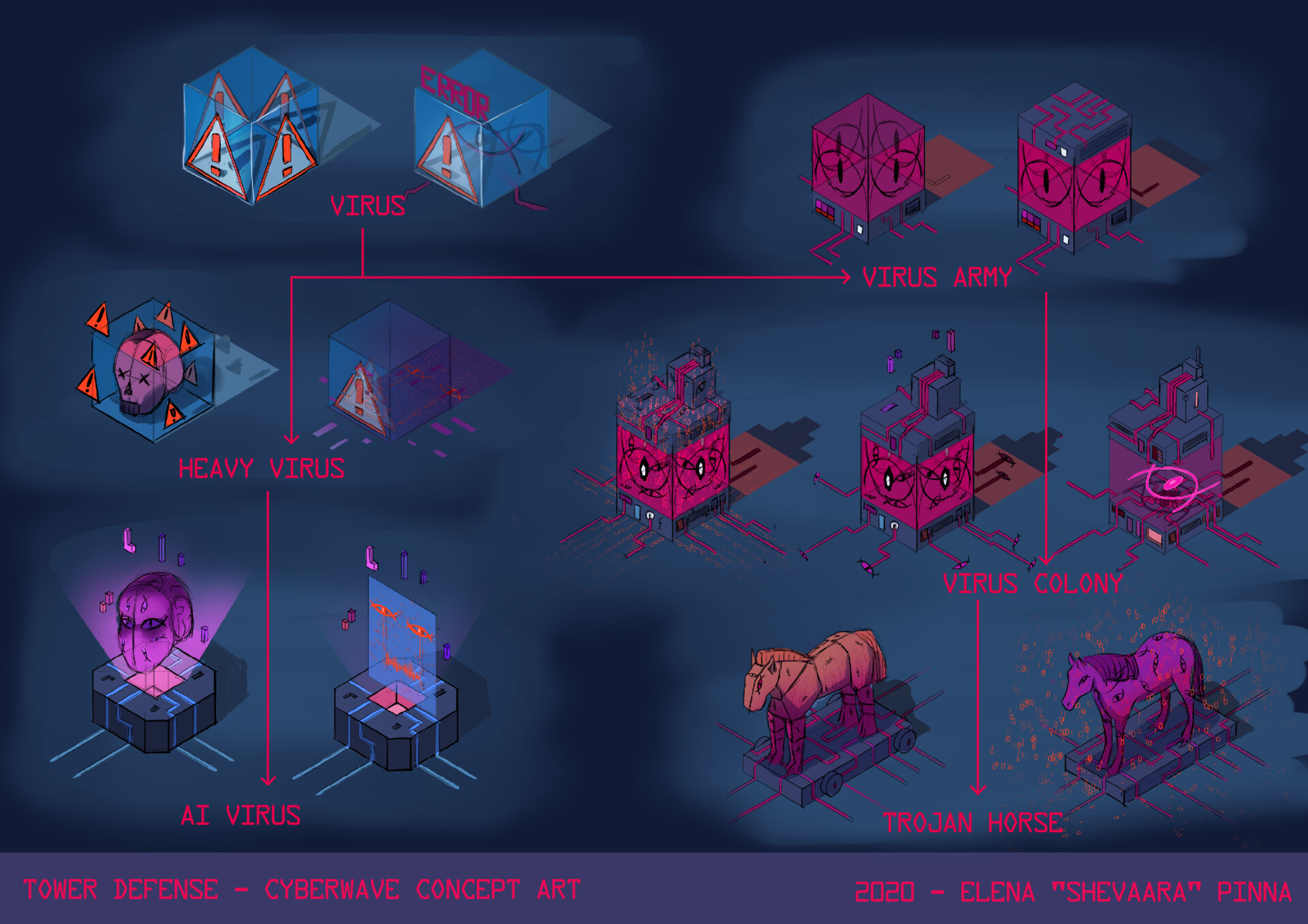The image is a digitally designed piece of concept art for a tower defense video game, titled "Tower Defense - Cyberwave Concept Art", created in 2020 by Elena Shavara Pena. The background is a dark blue, contrasting with the predominantly pink-hued art that covers the lower portion. The caption and credits are written in pink letters. Centrally, various virus types are depicted in an organized grid-like fashion, with square boxes connected by electrical lines forming a network. 

Starting from the top, the labeled components are:

1. **Virus**: Featuring two cubes with orange exclamation marks inside triangles.
2. **Heavy Virus**: Situated beneath 'Virus', showing a skull with X-ed out eyes, surrounded by orange arrows and triangles with exclamation points.
3. **Virus Army**: To the right of 'Heavy Virus', displayed with interconnected pink squares.
4. **Virus Colony**: Positioned above 'Trojan Horse', consisting of a complex structure of interconnected pink cubes.
5. **Trojan Horse**: Contains an orangish-pink horse on the left and a pink-purple horse on the right, connected by an arrow from 'Virus Colony'.
6. **AI Virus**: Below 'Heavy Virus', depicting a head on a square box with holographic-like effects, and another box with two orange fish-like figures.

This structure appears to illustrate the different components and threats within the game's mechanics, offering a detailed visual and textual explanation of the gameplay elements.